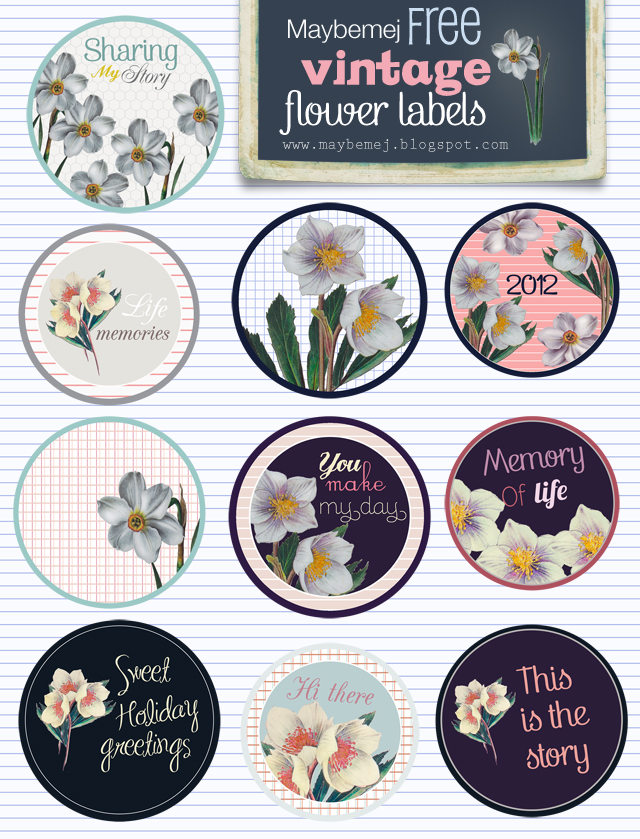This photograph features a collection of 10 vintage flower label stickers arranged in a 3x3 grid with one additional label at the top left. The background resembles lined paper, and in the upper right corner, the text reads "May Bembej Free Vintage Flower Labels" along with the URL "www.maybemedge.blogspot.com." Each circle contains a distinct flower design with varying colors including blue, pink, white, and yellow. Some of the labels include phrases such as "sharing my story" alongside white lilies with yellow centers, "life memories" with white flowers, "you make my day," and "sweet holiday greetings." Other labels are adorned with flowers and the years "2012," expressing sentiments like "memory of life," "hi there," and "this is the story." Notably, one segment of circles includes a combination of white and red flowers, adding diversity to the floral patterns. The different typefaces and colors enhance the visual appeal of these nostalgic flower labels.